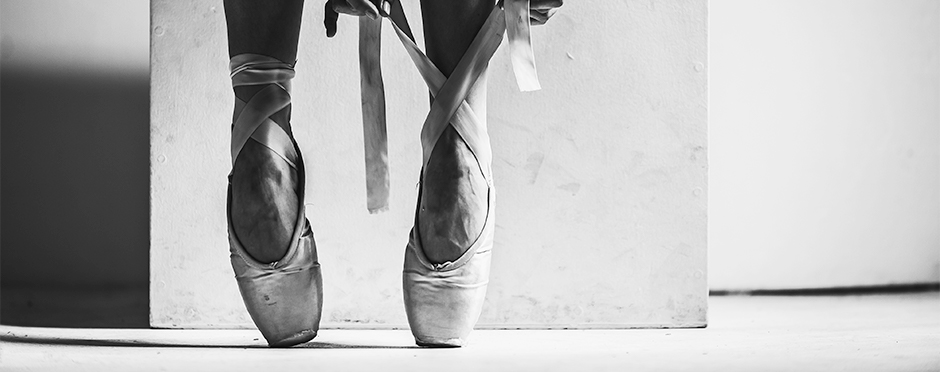In this striking, monochrome photograph, the focus is on a ballerina’s feet and ankles as she ties the laces of her worn, silverish pointe shoes. Captured in black and white, the image reveals the aged and beaten-up condition of the ballerina shoes, enhancing the raw, authentic feel of the composition. 

Her left foot, positioned slightly off-center to the right, is in the midst of being laced, while her right foot, already tied, stands poised on her tiptoes, projecting her shadow from right to left on the floor. The backdrop consists of layers: a predominantly white background with a darker, shadowed area on the left side, and a bright, rectangular block situated in the center. The photograph, elongated in shape, gives an intimate glimpse into the delicate yet demanding world of ballet, capturing both the grace and grit of the dancer.